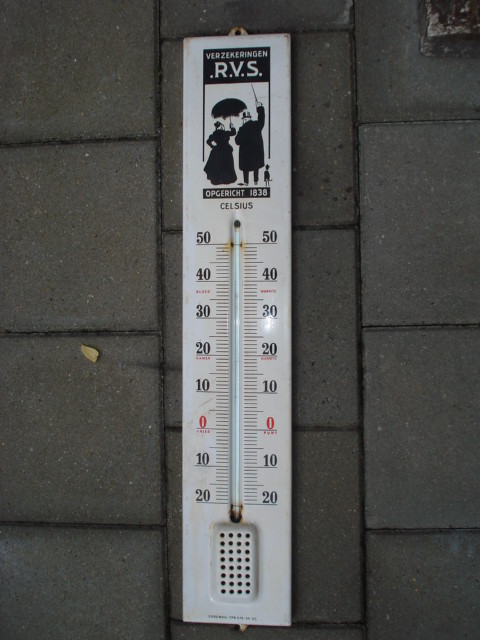This is a portrait-mode photograph of an outdoor thermometer mounted on a concrete tile surface. The thermometer itself is a long, rectangular, metal device painted white and centrally positioned within the frame. A small hanging loop is located at the top center for mounting. 

The thermometer features an intricate design at the very top, with a black-bordered, banner-like motif that reads "Verzeckringen RVS." Flanking the banner are two poles that add to its ornate appearance. Beneath this banner, the design portrays a woman dressed in an old-fashioned long dress, holding a parasol over her head. Positioned to her right is a man in a long black overcoat, black pants, black shoes, and a top hat, seen from the back. He holds a cane aloft with his right arm, directing attention towards the top center of the thermometer.

Below this illustrated scene, another black border reads "Opgericht 1836" or possibly "1838," though the exact year is unclear. The temperature is measured in Celsius, with numerical indicators running down both sides of the instrument. The thermometer itself is centrally situated within the metal mount. At the bottom of the device, there is a rectangular section featuring linear holes.

Overall, the thermometer’s historic and decorative elements, coupled with its practical function, are meticulously captured in this detailed, centered photograph.